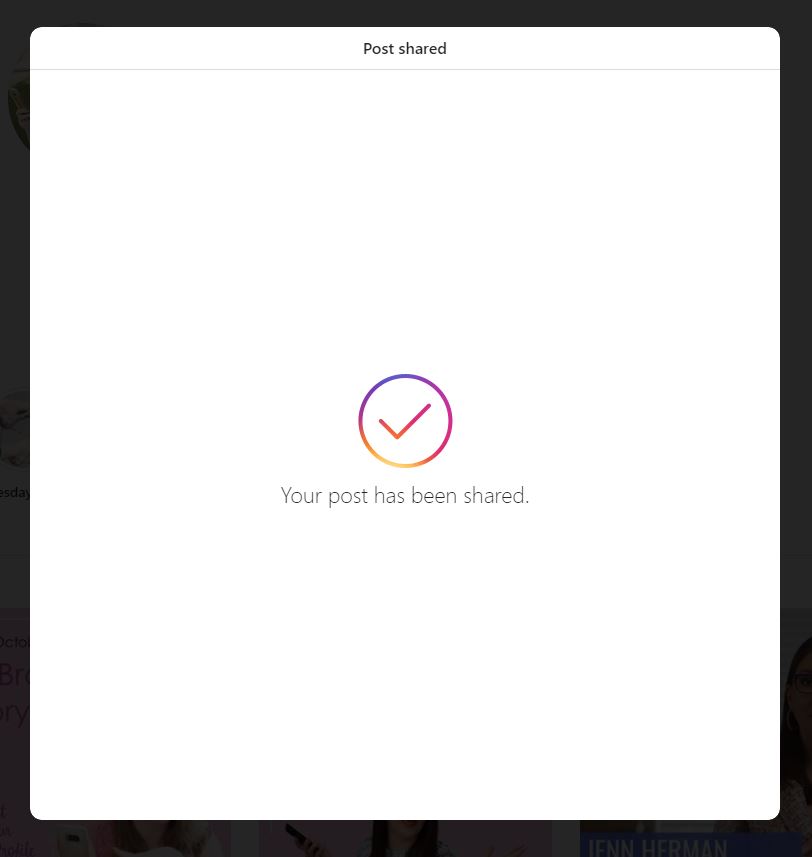Screenshot from Instagram on a Tablet – This image falls under the "Website Screenshots" category and features a confirmation screen from Instagram. The background is entirely white. At the very top, "Post shared" is displayed in small, black font, underlined in gray. Dominating the center of the page is a large checkmark filled with Instagram's signature gradient of blue, purple, yellow, and orange. Below the checkmark, the message "Your post has been shared" appears in gray text. This familiar screen appears whenever users share a post on Instagram. Judging by the dimensions of the screenshot, it was likely captured from a tablet, as it is too wide to be from a phone but not wide enough to be from a laptop.